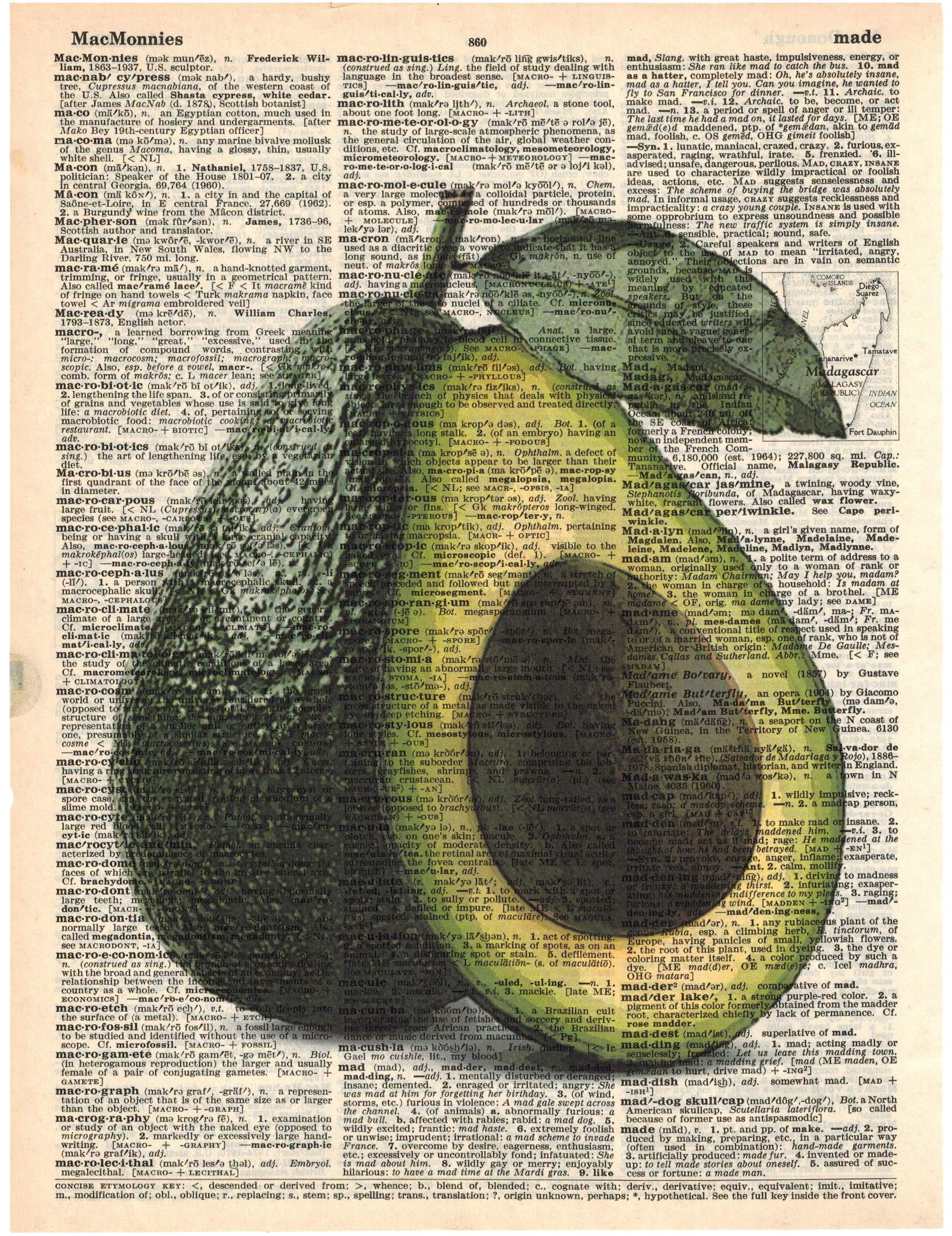The image displays a yellowed page from a dictionary, specifically page 860, spanning entries from "MacMoneys" to "Made." In the upper right quadrant of the page, there is a small image or map of Madagascar. Superimposed on this dictionary page is a translucent, color photograph of two avocados. The first avocado, positioned on the left, is whole with a green, bumpy surface, a visible stem, and a leaf at the top. In front of this whole avocado is a sliced half avocado displaying its yellow-green flesh and a prominent black pit. The translucent nature of the avocados allows the underlying text of the dictionary entries to be seen through the image, merging both textual and visual elements in a striking juxtaposition. The overall effect is both curious and detailed, blending elements of language and nature on a single aged page.